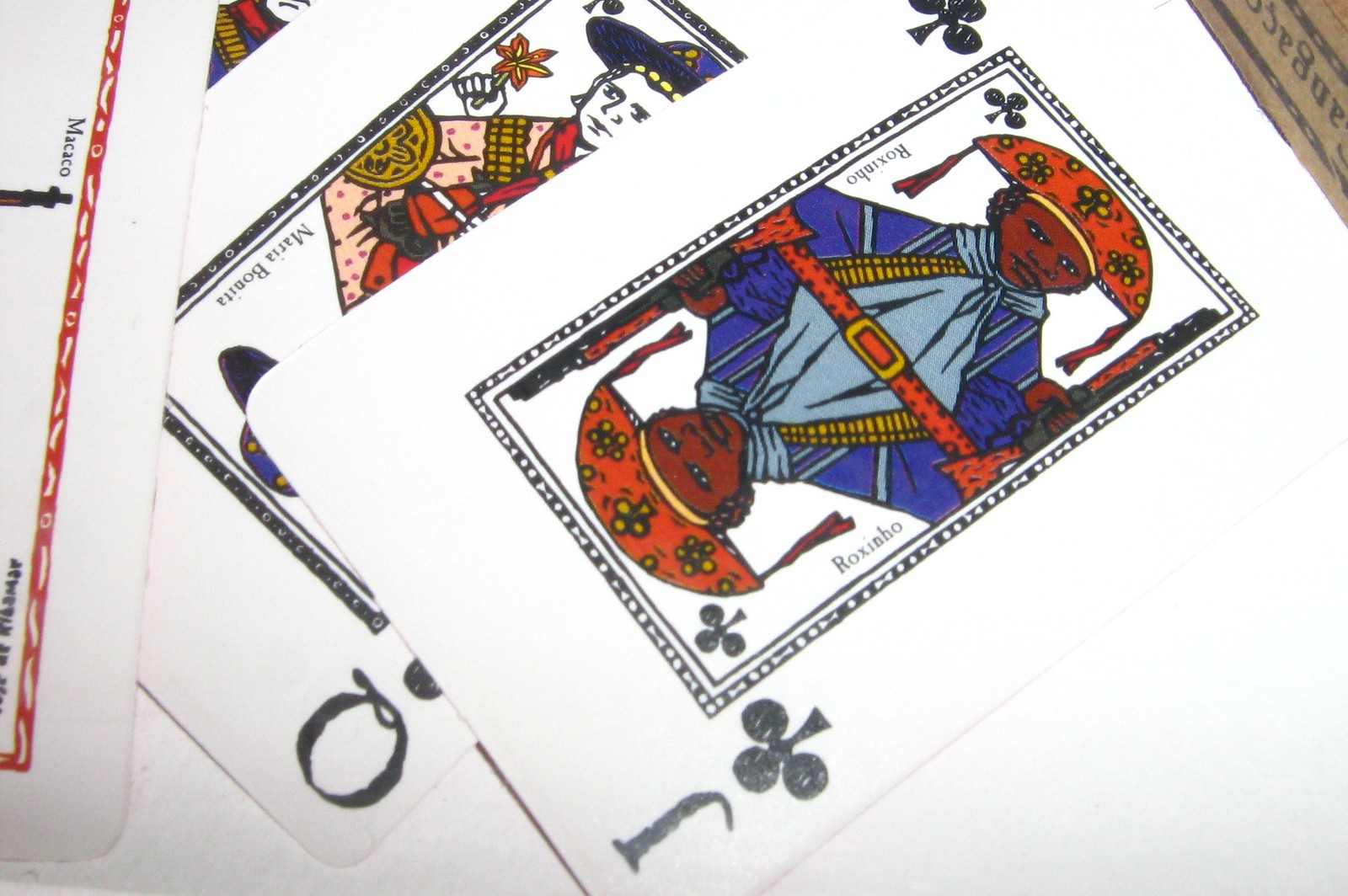The image showcases a close-up of four fanned-out playing cards against a pristine white background. In the top left corner, a small piece of brown cardboard peeks into the frame, featuring two black stripes with some letters nestled between them.

The primary focus is on the playing cards, which are thin and rectangular, arranged in a slightly messy but visually appealing pile. The foremost card is a Jack of Clubs, adorned with clubs in the top left and bottom right corners, alongside the letter 'J'. Central to this card is a mirrored image of a figure inside a black rectangle. The character wears an orange half-circle hat decorated with yellow clubs, a blue coat paired with a yellow sash, a green scarf, and an orange belt with a yellow buckle. This belt is the point of symmetry, dividing the mirrored images of the same figure, who appears to hold a cylindrical brown and black object, presumably a gun.

Behind the Jack of Clubs, another card partially reveals its features. A 'Q' indicates it is the Queen of Clubs. This figure dons a blue hat, a peach coat, and also sports a yellow sash identical to the Jack's. The Queen holds a coin in one hand and a flower in the other.

The final two cards in the composition are barely visible, with one showing slivers of yellow, red, and blue, and the other just a hint of a red line along the very left edge of the image.